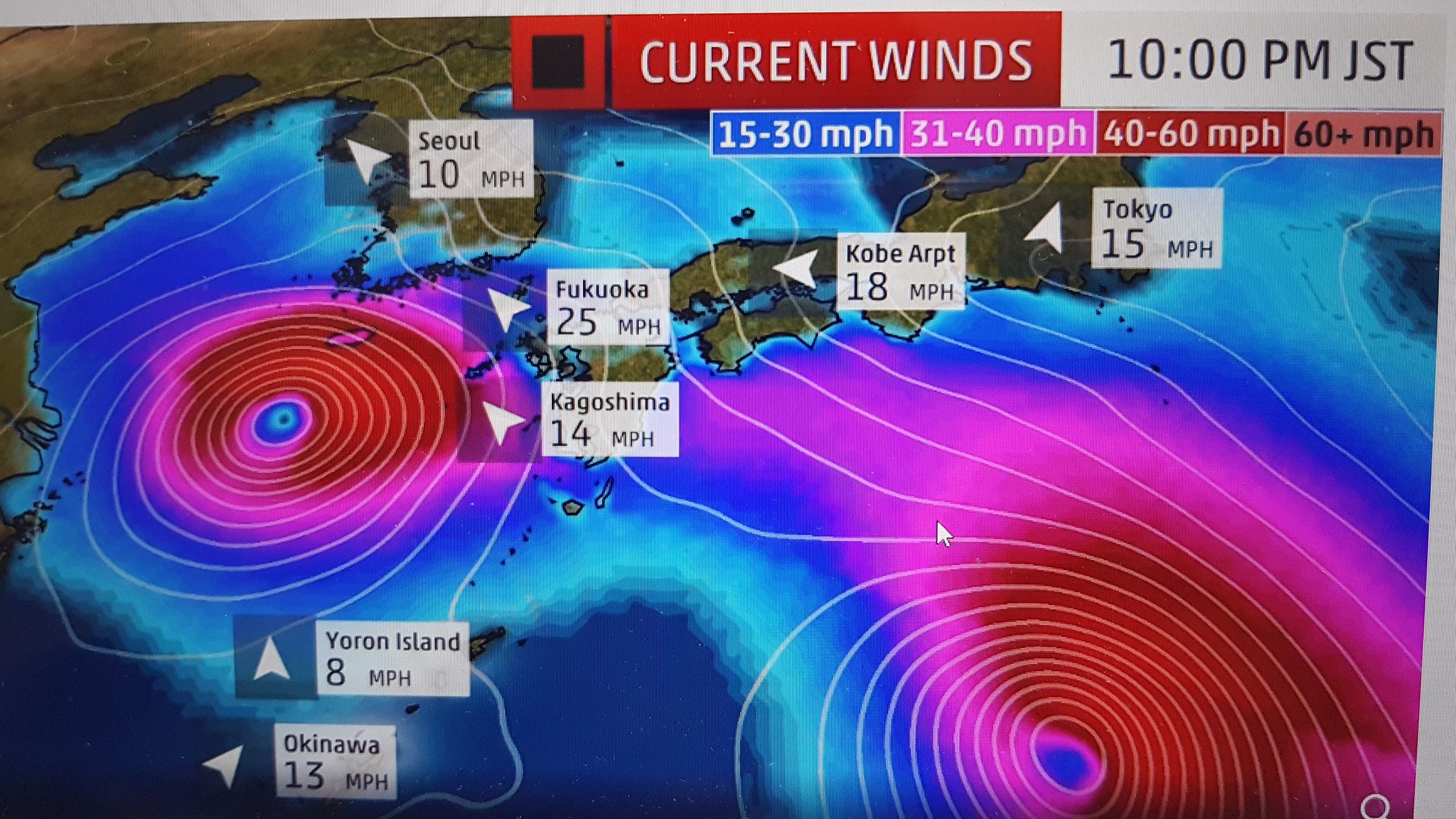This image is a screenshot from a television weather report centered on Japan, showcasing current wind conditions at 10:00 PM JST. In the upper right corner, a red rectangle contains the white text "Current Winds," while next to it, a white rectangle displays "10:00 PM JST" in black font. A color-coded legend beneath these labels details wind speeds: blue represents 15-30 MPH, pink is for 31-40 MPH, red indicates 40-60 MPH, and orange signifies winds exceeding 60 MPH. The main part of the image features a 3D map of Japan, overlaid with multiple lines directing towards the island, highlighting wind speeds in various locales. Specific velocities are noted: Seoul reports 10 MPH, Fukuoka 25 MPH, Kagoshima 14 MPH, Yoron Island 8 MPH, Okinawa 13 MPH, Kobe ARPT 18 MPH, and Tokyo 15 MPH, each marked with arrows pointing in various directions. The colored regions on the map correlate with the legend, visually representing the indicated wind speeds.